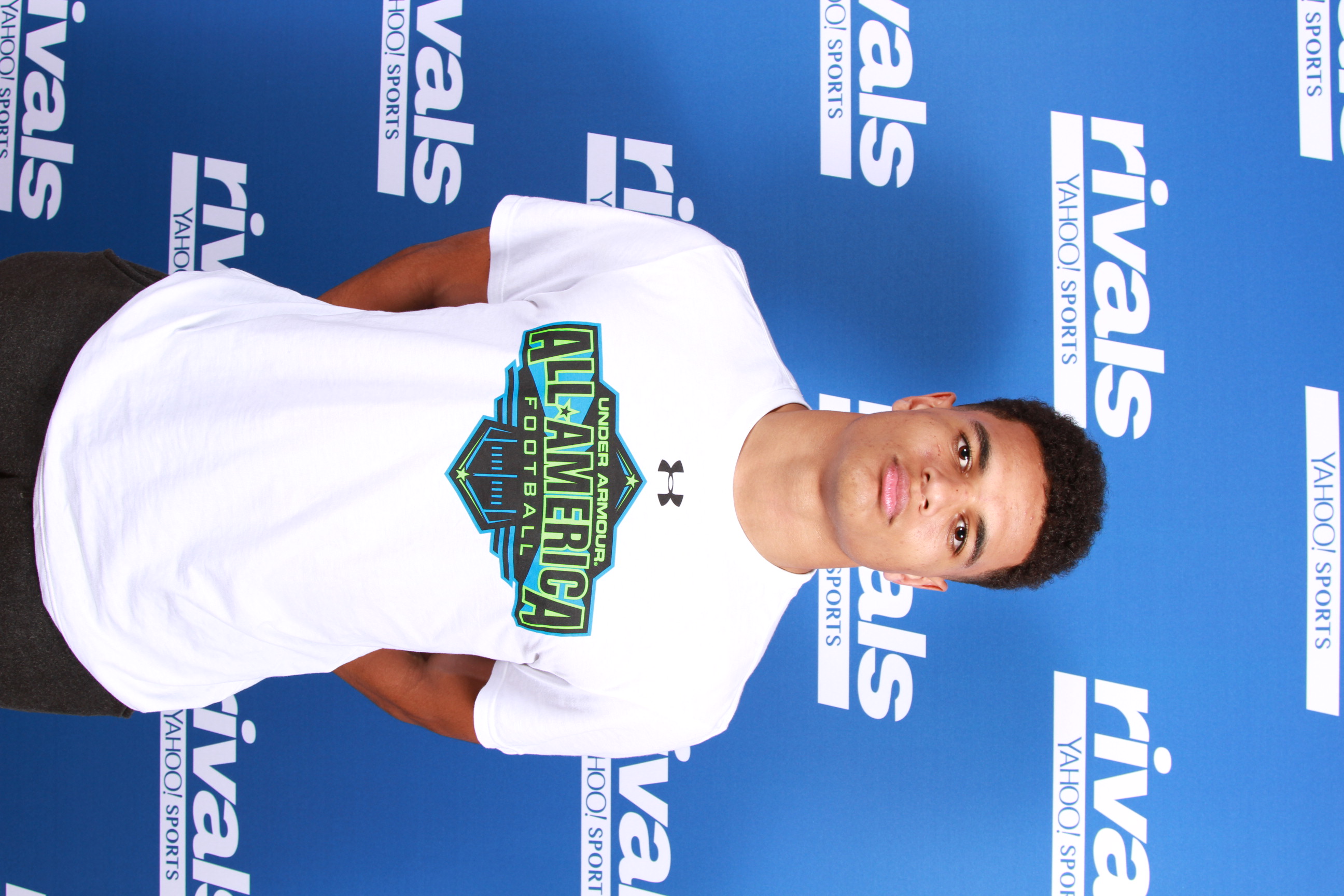This photograph, taken indoors in portrait orientation but displayed horizontally, features a young, light-complected African American man who appears to be in his late teens or early twenties. He possesses short, curly black hair and wears a white short-sleeved T-shirt adorned with the Under Armour logo and the words "Under Armour All-America Football" in black and light green letters. The young man stands with his arms folded behind his back, striking a stance suggestive of a formal or promotional photograph, possibly related to football. His expression is serious and composed, with his lips closed and chin slightly raised, conveying a sense of pride. He is dressed in black or possibly gray pants. The backdrop is a repeating pattern of the "Rivals Yahoo Sports" logo against a blue background, highlighting the sports-related context of the image.